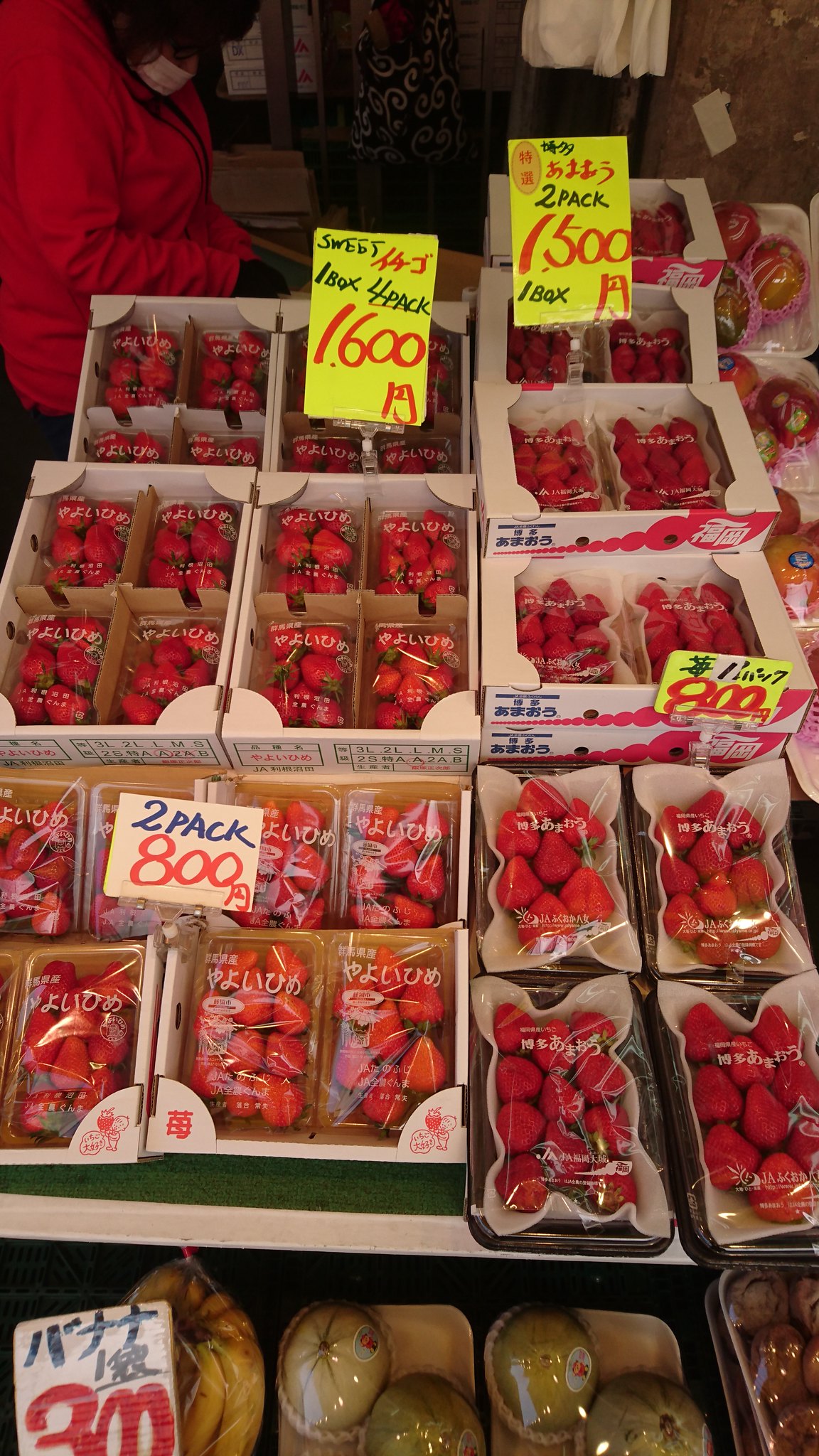This color photograph captures a bustling open-air market stall, likely set in an Asian or East Asian country, identified by the foreign script on the price labels. The focal point of the stall is the array of beautifully displayed, bright-red strawberries, all meticulously wrapped in plastic. The strawberries are sorted into various types of packages, including a two-pack, four-pack, and a singular pack, with prices such as 1,600, 1.5, 800 clearly marked on signs. Cardboard boxes prop up the produce, enhancing the rustic market vibe. 

In the colder weather, evidenced by her attire, a woman in a red long-sleeve jacket and a face mask, possibly a market vendor or a customer, stands towards the back, attentively examining the items on display. Her dark hair is noticeable against the colorful background of the market. Additionally, to the side and partially in the background, there's another individual in a black and white top with swirling patterns.

At the bottom of the image and to the left, other types of fruit can be seen, albeit also wrapped in plastic. There appears to be a variety of items including what looks like bananas and possibly green giant limes, adding more vibrant colors and diversity to the market scene.